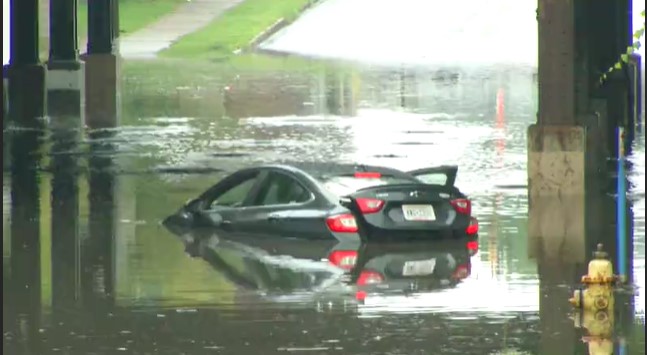A rectangular photograph captures the harrowing aftermath of an outdoor flooding event. At the focal point of the image, a small car, nearly submerged up to the edge of its front door, appears to be adrift in floodwaters with its trunk and passenger doors conspicuously open. The vehicle seems precariously suspended in the water, indicating recent, substantial rainfall. 

In the background, the water extends up a street, which dips beneath a bridge, evidenced by visible bridge pillars flanking the scene. Parts of the street remain above water, suggesting a low-lying area prone to flooding. Additionally, a fire hydrant protrudes from the water in the foreground to the right, highlighting that the inundated section is relatively contained yet sufficient to immobilize the vehicle.

The bright daylight, indicative of a clear sky, illuminates the scene, enhancing the stark contrast between the dry areas and the flooded street, and casting light on the severity of the flooding. The photograph poignantly captures the vulnerability of urban areas to sudden, heavy rainfall and the resultant flooding.